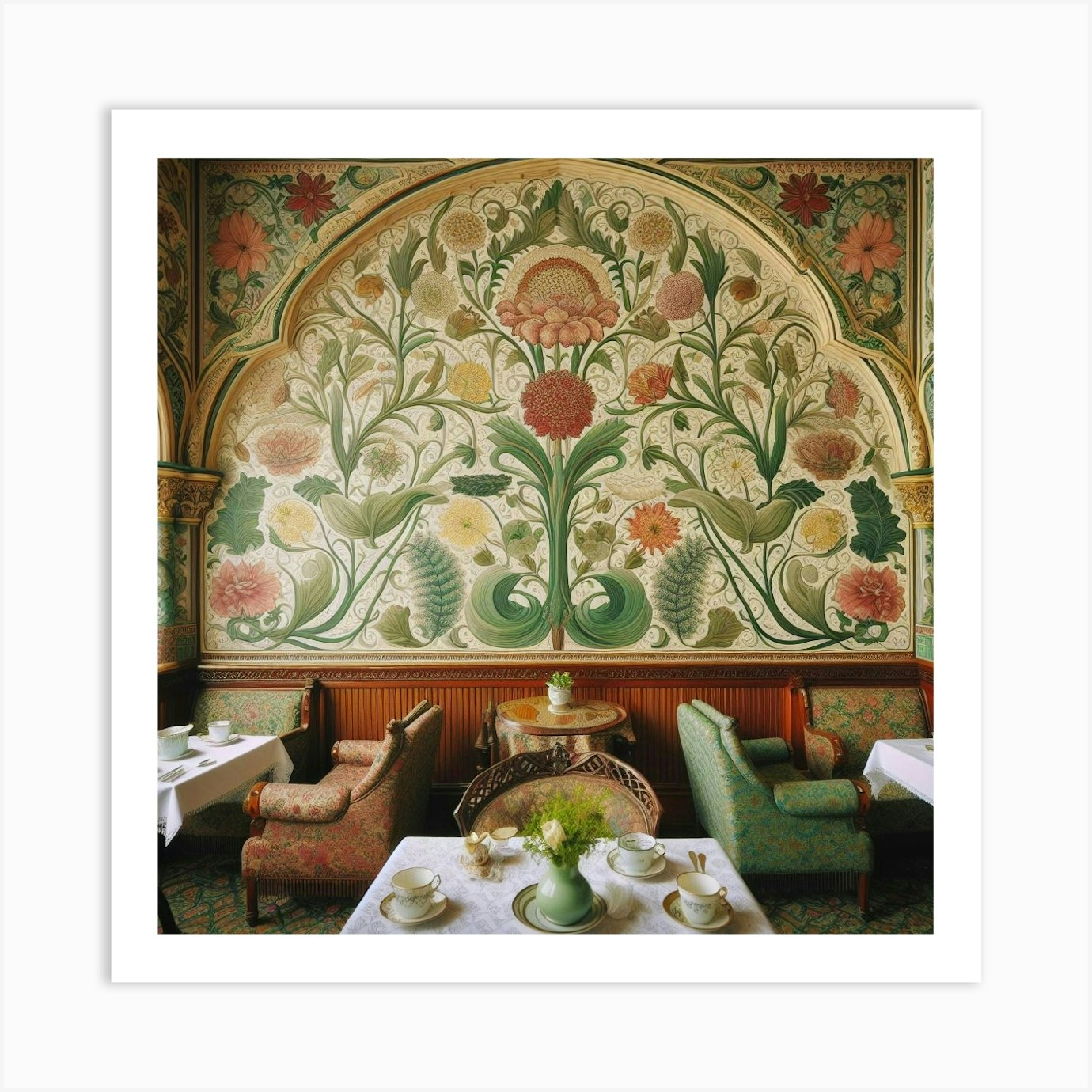This is an image of a beautifully decorated restaurant interior, possibly an art print or photograph, showcasing an arched back wall adorned with intricate floral patterns. The wall has a central motif featuring green stems and pink flowers set against a very light yellow background, which has gone through a shadowing effect giving it depth. The wallpaper extends to the upper right and upper left sections, interwoven with pink and red flowers on a greenish backdrop, almost resembling a tapestry. Near the base of this arched wall, the wainscoted lower portion adds an elegant touch. The restaurant is furnished with several tables: in the left and right corners are small tables with white tablecloths and fabric armchairs, complete with place settings. Centered in the image is a small round table with a plant, and in the forefront, there's a small white square table with a vase of flowers and more place settings, accompanied by a wicker-backed chair. The overall setting is refined, with impeccable detail in the furnishings and ornamentation, making it inviting and meticulously arranged.